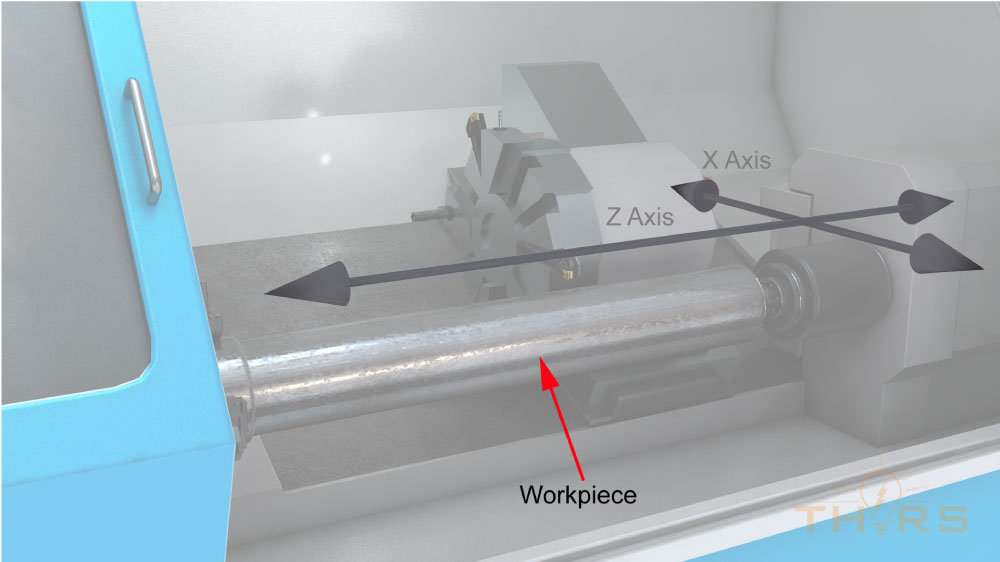The image presents a detailed schematic of a machine turning tool, primarily in black and white with distinct blue elements. Central to the schematic is a cylindrical steel rod labeled "workpiece," indicated by a red arrow. Positioned around the rod, there is a large screw-like mechanism at the core, and to its side, a component with a white roller. Two perpendicular black arrows labeled "X-axis" and "Z-axis" define the machine's spatial orientation. Prominently, on the left side, there is a blue door featuring a silver handle and a gray window. The blue door color is repeated subtly at the image's bottom, which is partially cut off. A watermark reading "Thor's" in yellow or brown is located in the lower right-hand corner. The overall layout lacks a specific background and is horizontally rectangular with no border, emphasizing the technical details for engineering purposes.